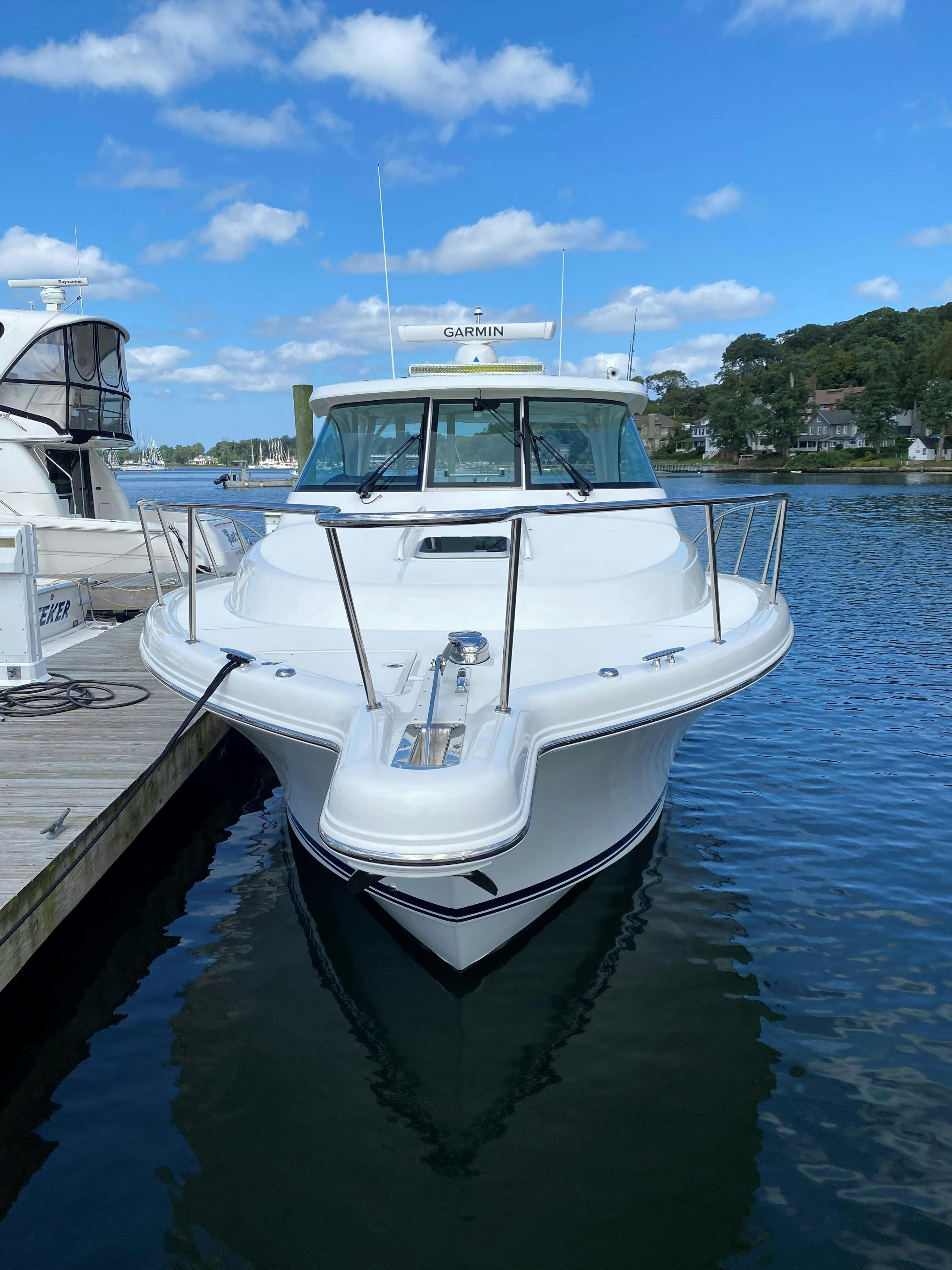This image captures a striking view of a white yacht docked at a marina on a clear day with a bright blue sky and a few clouds. The camera is positioned about 5 or 6 feet from the front of the yacht, offering a direct view of the vessel's nose. The yacht sits in dark blue, calm water with silver metal railings encircling its perimeter for safety. At the very front, there's a small, railed plank that can be used for spotting fish or harpooning. This one-story yacht, equipped for probably saltwater fishing, likely operates as a charter boat with a captain.

The central section of the yacht is an enclosed pilot house, which provides protection for the driver, featuring large windshields and windshield wipers to ensure visibility and safety during adverse weather. Atop this enclosed area is a rotating radar device branded with "Garmin," accompanied by at least two antennas, indicating a well-equipped navigation system. 

In the background, across the water to the right, you can see a grass-covered coast dotted with trees. Further across the water, there are visible houses and more docks, enhancing the picturesque setting. Additional boats are tied up at the dock, particularly on the left side where a two-story yacht is noticeable, contributing to the bustling yet serene atmosphere of the marina.